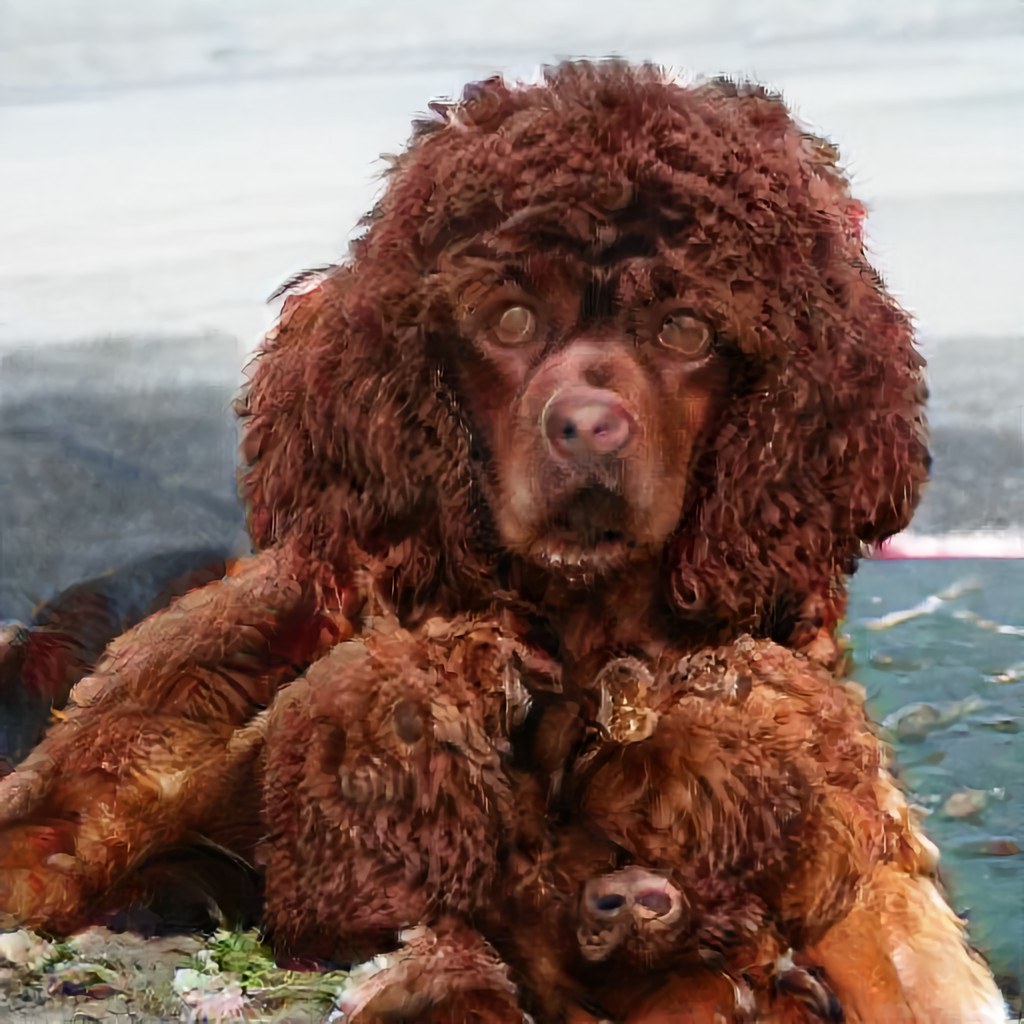The image depicts a creature resembling a dog with an overwhelmingly fluffy, chocolate-brown coat. Its head is crowned with afro-like, poofy hair and distinct, floppy ears. The creature's eyes are a lighter brown, exuding a slightly hazy and sorrowful expression, and its nose appears somewhat disfigured, blending shades of brown and pink. The body is adorned with an abundance of fluffy hair, extending prominently from the chest area. On closer inspection, the lower part of the body seems peculiar, with multiple dog-like noses and eyes jutting out at odd positions, enhancing the uncanny valley effect that hints at an AI-generated origin.

The background features a mix of natural elements, with a grayish sky possibly accompanied by clouds, and glimpses of what appears to be ocean or water on the right side. A dirt patch and grassy terrain can be observed in the foreground, giving the scene an eerie, surreal feel. Overall, the image combines elements of realism and oddity, making the creature's appearance seem both familiar and disturbingly distorted.